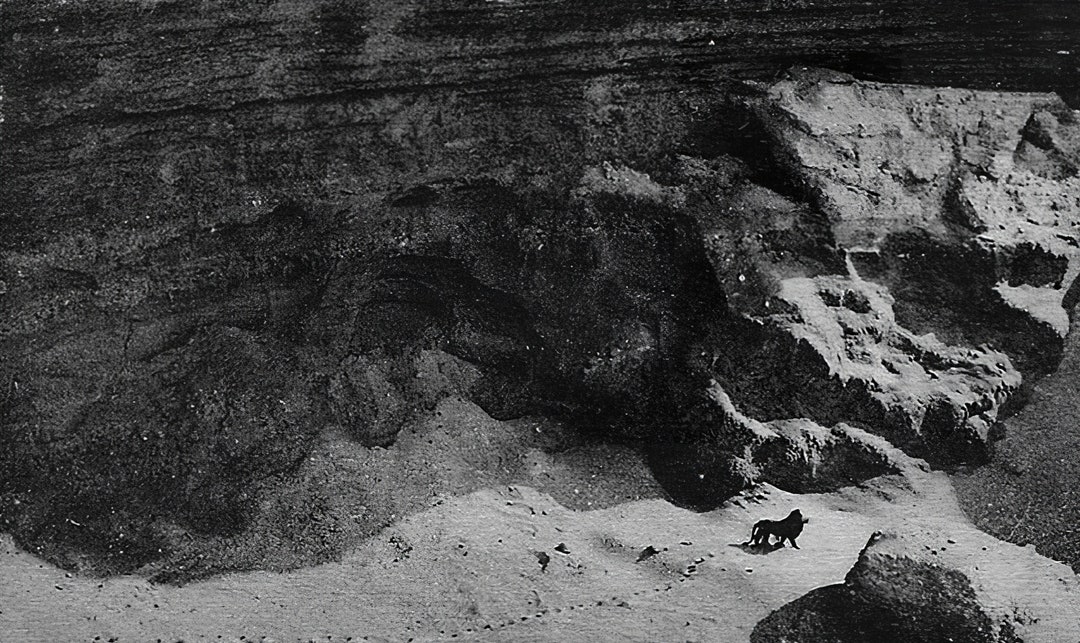The image appears to depict a vast, sandy canyon with towering rock walls that stretch all the way to the top of the frame, curving inward to give the impression of a cave entrance. The scene is monochromatic, possibly black and white, contributing to an overall stark and desolate atmosphere. In the foreground, footprints in the sand lead up to a solitary animal, which seems to be a lion, though its exact species is ambiguous due to the blurry quality. The left side of the canyon is slightly darker, while the right side appears lighter, suggesting that natural light is filtering through a cave mouth. The rock formations exhibit distinct layers, enhancing the geological impression of a valley or canyon. The scene lacks any additional elements such as trees, water, or other animals, adding to its dramatic and isolated feeling. The image's appearance—potentially either a real photograph or a CGI creation—evokes a sense of wilderness and untamed beauty.